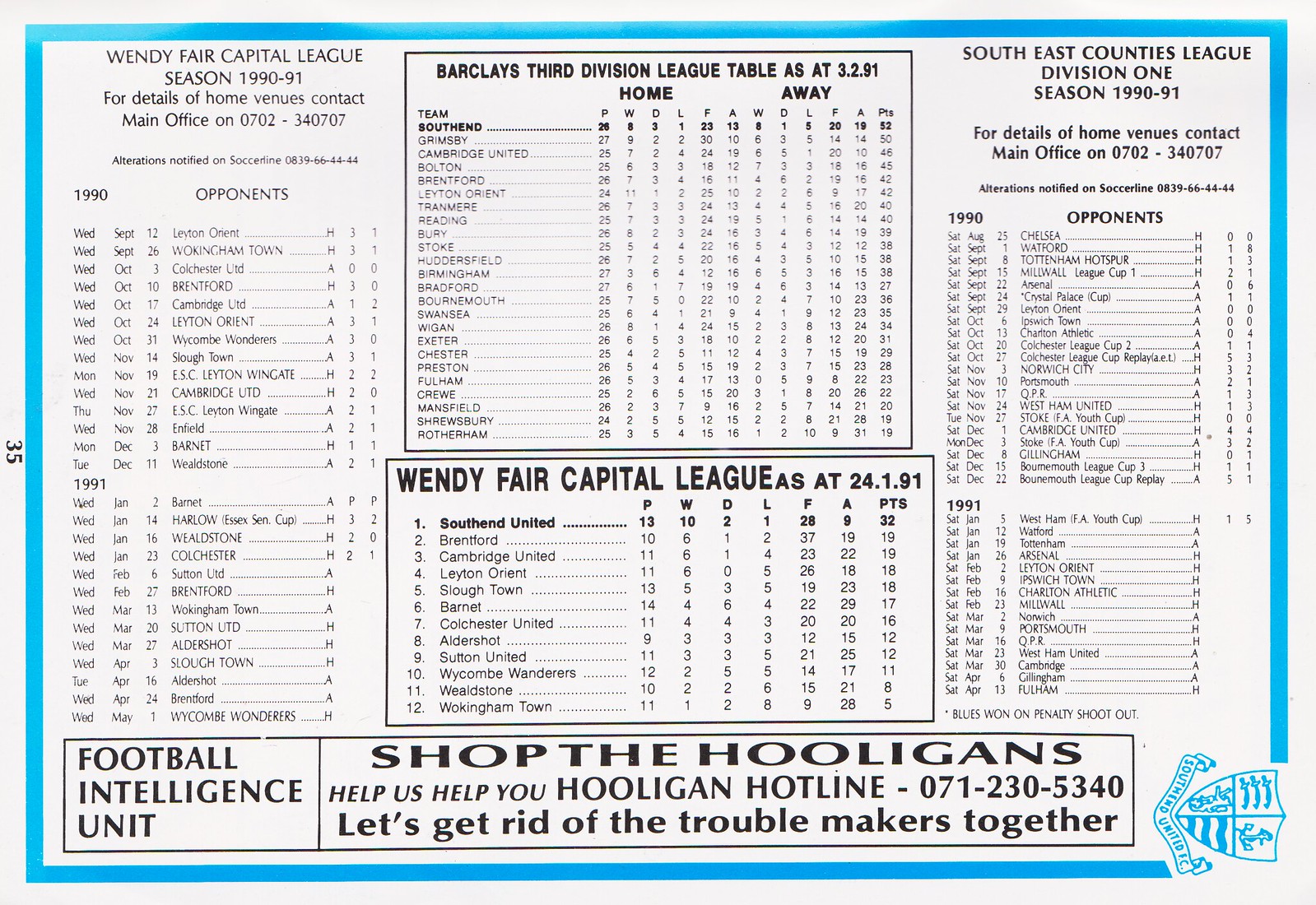This image is a horizontally oriented page with a light blue border, resembling a statistical schedule from a sports league program, specifically related to football. At the top left, it reads "Wendy Fair Capital League, Season 1990-1991," followed by details such as opponent names, dates, and scores, organized into columns for the years 1990 and 1991, with only a few results recorded for 1991. In the center, a prominent black-outlined box titled "Barclays Third Division League Table as of 3-2-91" displays various statistical standings, including home and away records. Below this is another black-outlined rectangle providing a summary for the Wendy Fair Capital League as of 24-1-91, listing 12 teams and associated player statistics. On the far right, the column header "Southeast Counties League Division I, Season 1990-1991" introduces a similar listing of opponents and match results for the years 1990 and 1991. The bottom of the image features a long black rectangle, left-aligned with the text "Football Intelligence Unit" and "Shop the Hooligans," including a hooligan hotline number for reporting troublemakers. The bottom right corner bears an emblem resembling a coat of arms. Additionally, a small page number "35" is printed along the left side, suggesting this page is part of a larger landscape-formatted document.